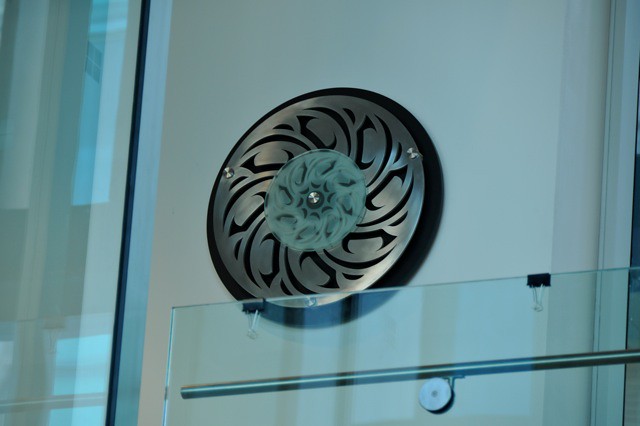The photograph captures a detailed view of a distinctive metal object mounted on a plain white or off-white wall. The centerpiece of the image is a round metal disc with intricate designs, including C-shaped and linear cutouts. This disc is primarily silver and features a light sea green or sage green translucent middle section, resembling a pinwheel, secured by a central metal rivet. Surrounding the central plate is a copper-colored ring with three visible rivets—at the top, left, and bottom—securing the disc to a slightly larger black border. 

In the background, we can discern additional elements that add context to the scene. To the left, partially visible through reflections on a glass surface, appear to be metal beams descending vertically, accompanied by a black line that runs the length of the glass. The background wall features a closed window with its curtains drawn. Additionally, the image hints at a railing or handrail attached to a glass partition at the bottom, suggesting the area might be on an upper floor. Two black paper clips with silver looping handles are fastened to the top of this glass panel, adding a final touch of detail to the setting.